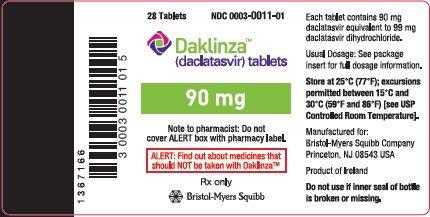This image features the label of a medication product, designed in the style typically found on a pill bottle or medication box. The background is white, providing a clean canvas that highlights various elements on the label. Along the left margin, a vertically-oriented UPC barcode is prominently displayed, with corresponding numerical digits underneath.

To the right of the barcode, the medication's name and logo catch the eye. The logo consists of a diamond shape with an intricate design of swirling purple and green colors. The name "DAKLINZA" is prominently printed in lime green, accompanied by the trademark symbol "TM" in the same color. 

Beneath the primary name, the text "DAKLATACIVIR Tablets" is shown, clarifying the medication's specific type. Directly below this, a vivid green banner stretches horizontally across the label, with the dosage "90 mg" boldly stated in white text.

On the far right side of the label, an important notation provides further detail about the medication's composition: "Each tablet contains 90 mg DAKLATACIVIR, equivalent to 99 mg DAKLATACIVIR dihydrochloride."